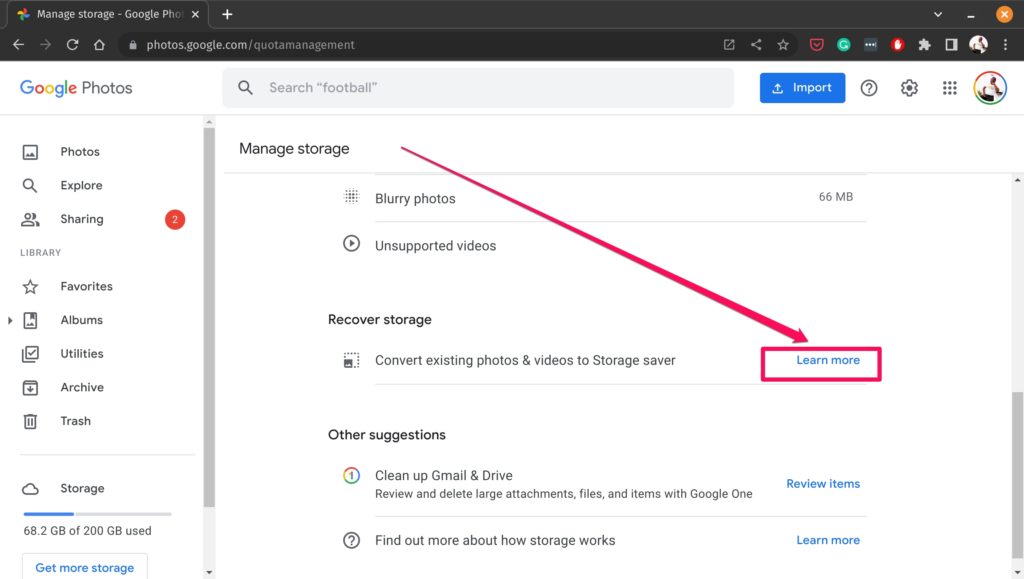This is an image of a screenshot, likely taken from a web browser resembling Google Chrome. At the top, the browser's tab bar indicates an open tab titled "Manage Storage - Google Photos," with a close ("X") button and a "+" button for adding more tabs. The upper right corner features minimize and close buttons typical of Chrome's interface.

Beneath the tab bar, there is a navigation toolbar with back, forward, refresh, and home buttons. The URL in the address bar reads "photos.google.com/quota management," and beside it are share and favorites buttons, along with various browser extension icons.

The central portion of the screenshot focuses on the Google Photos interface. At the top, "Google Photos" is labeled next to a search bar containing the phrase "search football." Adjacent to this is a blue "Import" button, followed by help and settings (cogwheel) icons, and a profile icon depicting a person in a white shirt.

The main content area displays storage management options. These include "Manage storage" with specific categories and their respective storage usage: "Blurry photos: 66 MB" and "Unsupported videos." Other actions listed are "Recover storage" and "Convert existing photos and videos to storage saver," each with a "Learn more" link marked by a pink arrow. Additional suggestions include "Clean up Gmail and Drive," "Review and delete large attachments," and "Files and items with Google One," with a "Review items" blue button. There is also a "Find out more about how storage works" link with a "Load more" button nearby.

On the left sidebar, navigation options are present: Photos, Explore, Sharing, Favorites, Albums, Utilities, Archives, and Trash. The storage usage is displayed at the bottom, showing "68.2 out of 200 GB used."